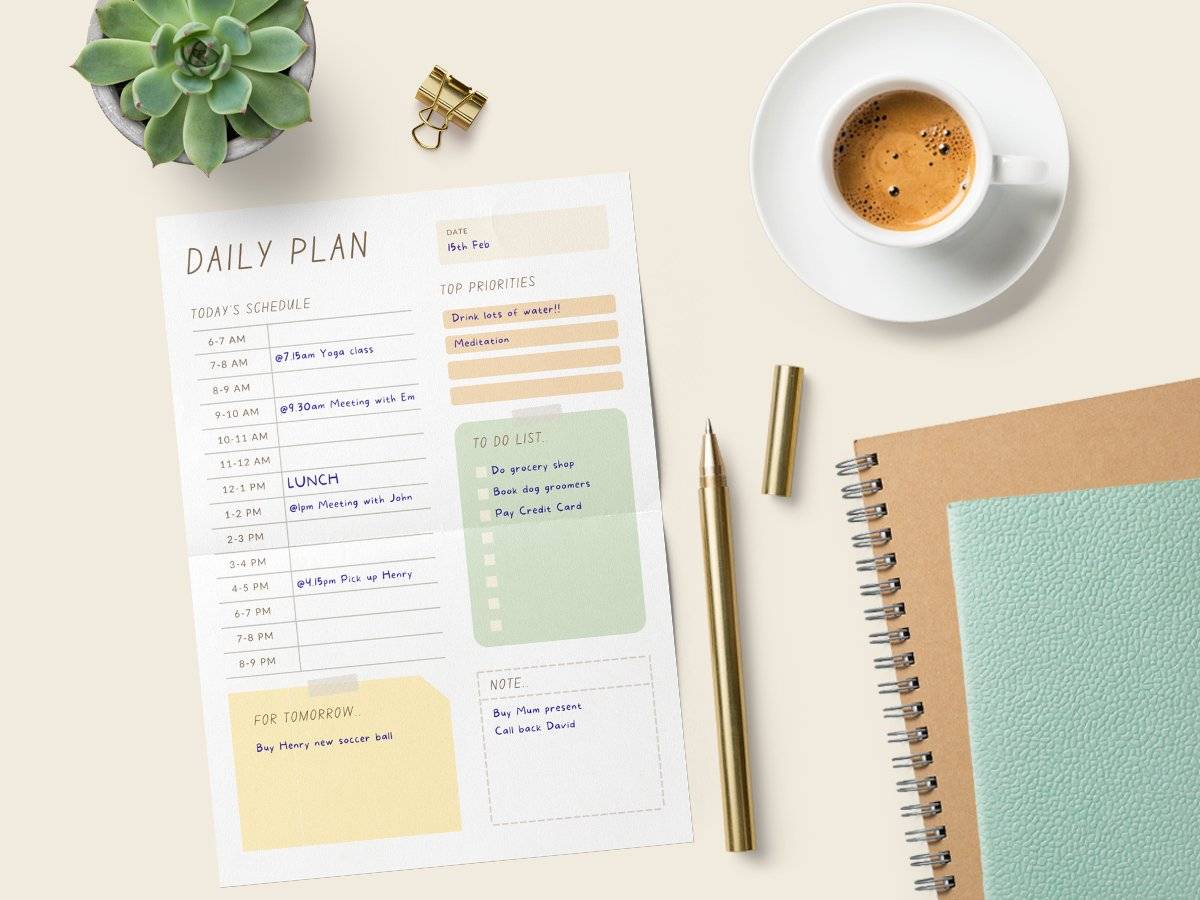A carefully arranged flat lay photo showcases a beautifully composed tabletop scene. At the center is a steaming, rich cup of coffee, topped with frothy, bubble-laden foam, suggesting a cappuccino or similar specialty brew. In the upper-left corner, a small plant with short, round, olive-green leaves—reminiscent of a medicinal plant—adds a touch of nature, housed in a sleek, gray flower pot.

Scattered around the table are various golden accessories: a paper clip, a spring clip, and an uncapped gold pen, imparting a feeling of opulence. Beside these items rests a daily planner, meticulously filled out with a myriad of tasks and appointments. The planner, marked for the 15th of February, includes a detailed schedule: "7:15 am Yoga class, 9:30 am Meeting with M, Lunch, 1:00 pm Meeting with John, 4:15 pm Pick up Henry, Buy mama present, Call back David, Do grocery shopping, Book dog groomers, Pay credit card, Drink lots of water, Meditation, and Buy Henry a new soccer ball," delineating a day packed with engagements.

In the lower-right corner, a spiral notebook is partly overlaid by a textured green folder, hinting at more written plans or notes. The tabletop itself, a very light off-white with a slight reddish hue, provides a warm and inviting backdrop to the scene.